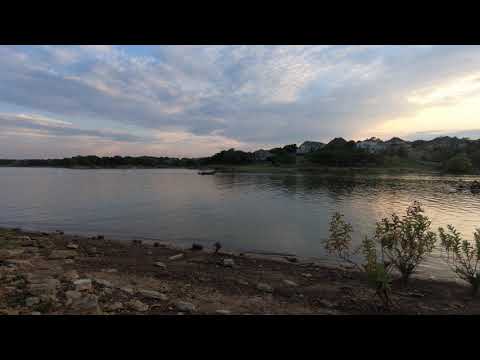This image, enclosed within thick horizontal black borders at its top and bottom, captures a serene lakeside scene bordered by trees. In the foreground, there's a rocky dirt shoreline sparsely covered with small plants and short bushes, leading to a calm expanse of water that stretches into the distance. Toward the center of the lake, a blurry silhouette suggestive of a kayak or canoe sits quietly on the water. Beyond the lake, on the far shoreline, more trees can be seen, with hints of rooftops peeking through, though they too are blurred. The sky dominates the upper portion of the image, showing a mix of bright white, feathery clouds interspersed with grayer, blanket-like clouds, with patches of blue sky peeking through. The illumination suggests it's either very early or late in the day, as the sun creates a bright reflection on the water’s surface, particularly noticeable on the right side. Detailed with a beautiful spectrum of colors—blue, gray, white, orange, yellow, black, and brown—this outdoor scene is tranquil and picturesque, encapsulated perfectly in a small square frame.